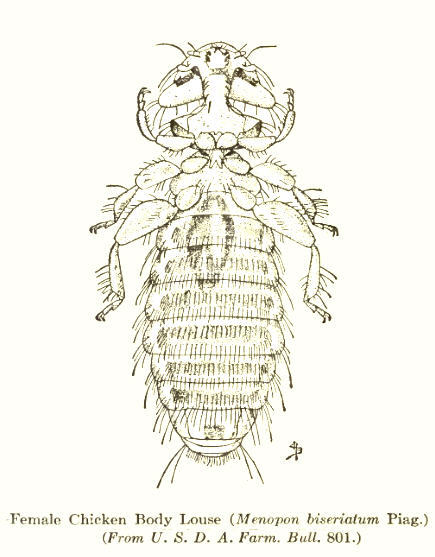The image is a black and white, hand-drawn illustration resembling a pencil sketch, set against a very light off-white background. It depicts an insect, specifically identified as a female chicken body louse, with distinct features including multiple oval sections and hair on its eight-part torso. The drawing has an intricate level of detail, suggesting it may come from an older book, reinforced by an older-style font and a slightly beige tone to the page. Below the sketch, black lettering reads "Female Chicken Body Louse" and in parentheses, "Menopon bisseratus." Additionally, there is a notation, "From USDA Farm Bull 801," and a small emblem located in the lower right section. The insect's detailed body, head, and legs are distinctly illustrated, giving it almost a lifelike appearance.